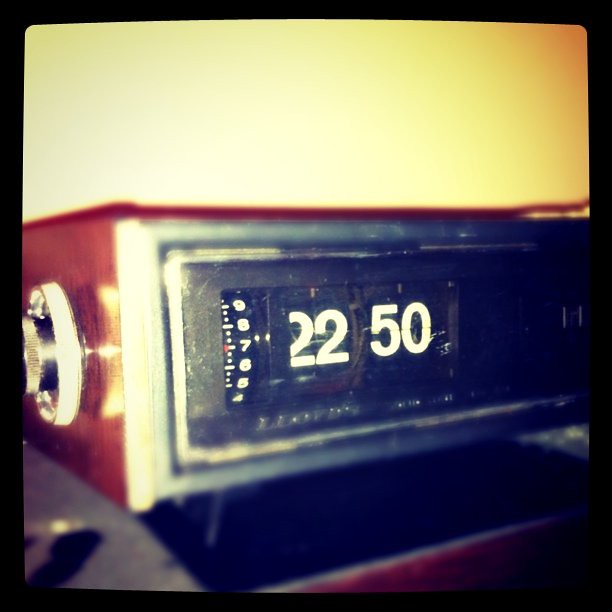This close-up image captures an old-fashioned alarm clock radio set to 22:50 (10:50 PM). The clock features a classic flip-style mechanism with black number plates and white numerals. Each number flips over individually, reminiscent of vintage card holders. The clock's face is adorned with a black background and is bordered by two concentric silver metal frames. 

On the left side of the clock's face, there's an additional dial marked with numbers ranging from 4 to 9, aligned vertically with horizontal lines and double dots between them, suggesting it might be the radio dial. Below the main time display, "Lloyd's" is visibly branded, indicating the manufacturer. 

Encased in either genuine or simulated mahogany wood, the clock has a silver metal knob on its left side with ridged edges for better grip, likely used for setting the time or tuning the radio. Though the surrounding elements are slightly out of focus, the clock rests on a gray counter with a wooden edge. A possibly yellow and grainy wall forms the blurry, rounded-corner background within the frame's black border, creating an authentic retro ambiance.